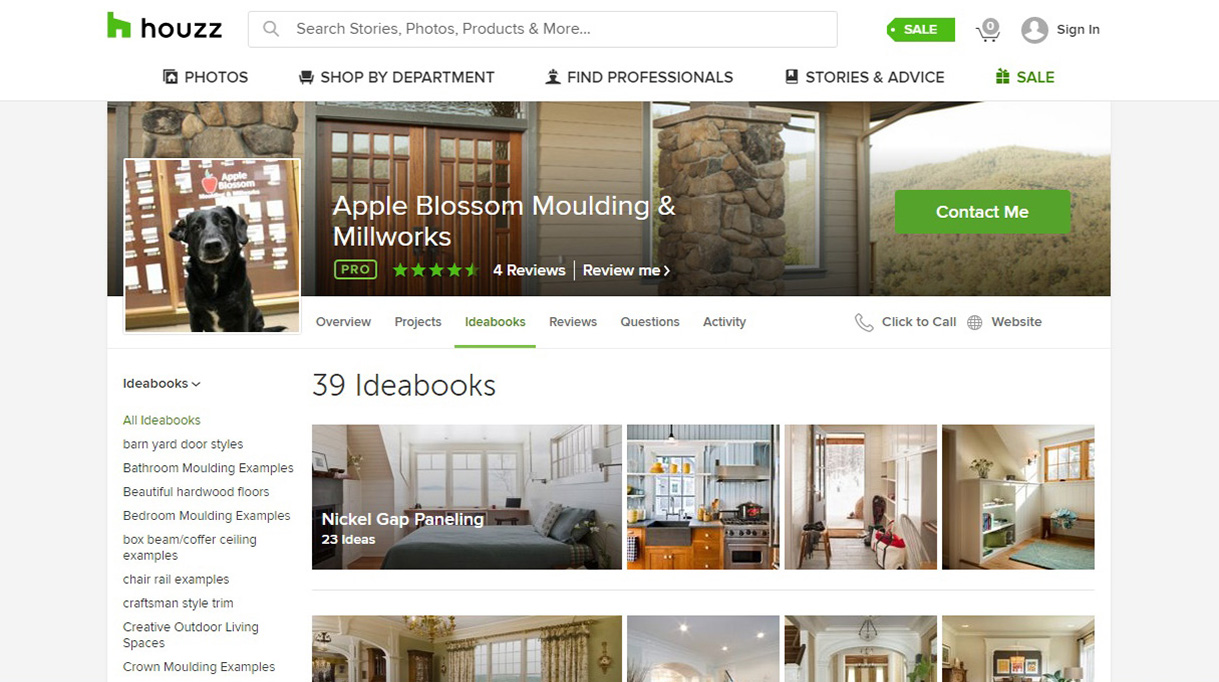A screenshot of the Houzz website showcases a meticulously designed interface with a white and lime green color scheme. At the top of the page, a search box invites users to explore stories, photos, products, and more, located next to a prominent lime green logo of a house in the shape of an "H." Adjacent to the search box, a 'Sale' button entices visitors with potential deals.

Dominating the upper left corner of the main content area, an image of a dog sits beside the title "Apple Blossom Molding and Millworks." The left-hand navigation menu lists categories such as "All Idea Books," "Barnyard Door Styles," "Bathroom Molding Examples," and "Beautiful Hardwood Floors," among others.

The centerpiece of the webpage displays 39 idea books, each represented by thumbnail images showcasing various interior designs. The highlighted idea book, "Nickel Gap Paneling," offers 23 creative ideas for its use. This website appears to be a home design service platform where users can browse design inspirations and possibly book services for their own projects.